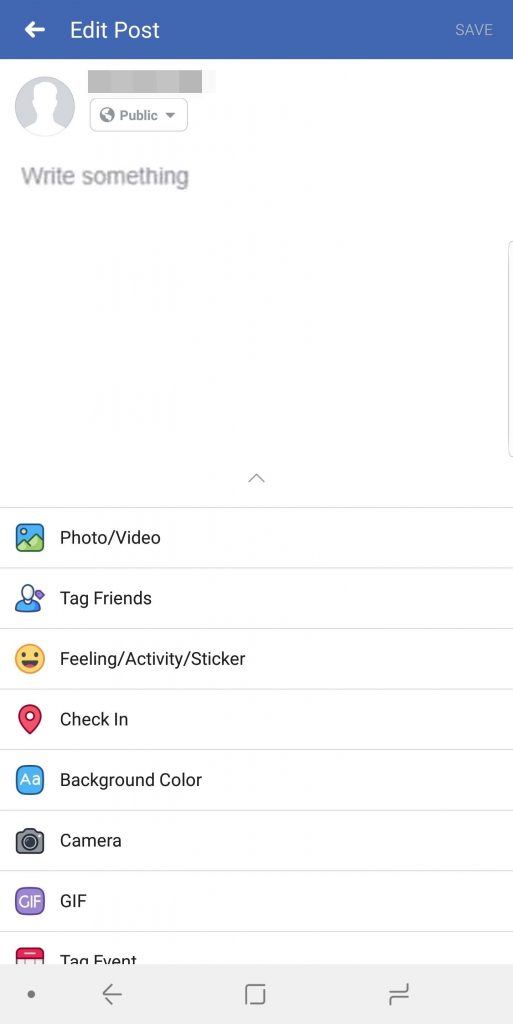The image appears to be a screenshot from a cell phone, specifically from a social media app's post editing screen. The interface is primarily vertical and rectangular. At the top, there is a blue bar with the words "Edit Post" displayed in white text, accompanied by a white left-pointing arrow. Below this bar, there is a circular icon featuring a default, all-white person silhouette, signifying a user profile. Adjacent to this icon, there is a box labeled "Public" with a downward-pointing arrow next to it, indicating the privacy settings for the post.

Beneath these elements, there is a prompt that reads "Write something..." followed by a large, empty white text box intended for the user to write their post. Under this text box, a series of options are displayed in a list format, each paired with an icon and descriptive text:

1. A photo icon accompanied by "Photo/Video"
2. A person silhouette icon with the text "Tag Friends"
3. A smiling emoji icon labeled "Feeling/Activity"
4. A red location pin icon next to "Check In"
5. A blue square featuring an uppercase and lowercase "A," labeled "Background Color"
6. A black camera icon with the word "Camera"
7. A purple square with the word "GIF" displayed on it

The bottom section of the image appears to be cut off, with partial visibility of another option.